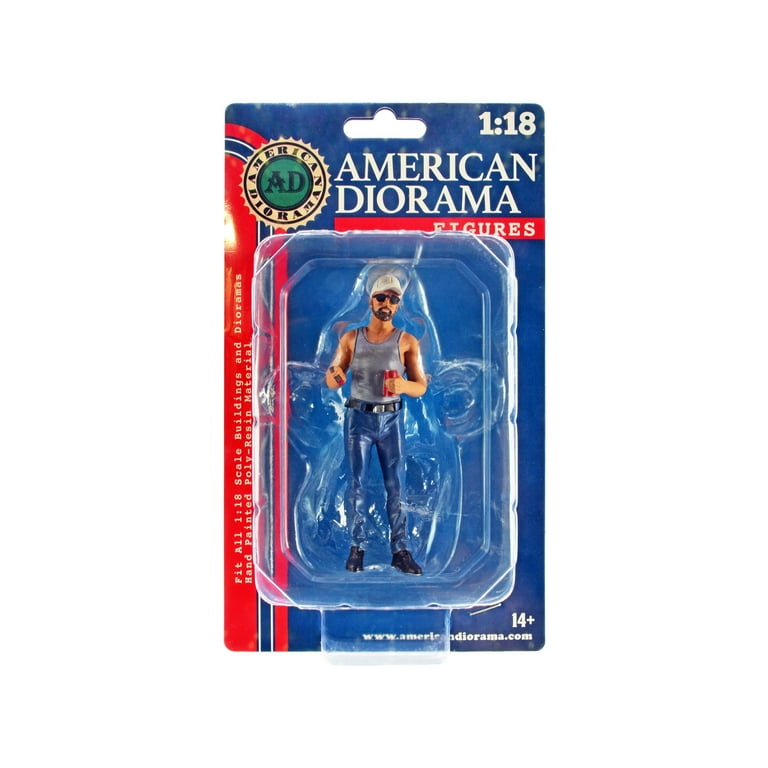The image depicts a detailed action figure encapsulated in its original, though somewhat worn, blister packaging against a plain white background. The top of the package prominently features the title "American Diorama Figures" alongside a circular emblem with a gear-like design, within which "A.D." and "American Diorama" are inscribed on a green background. The packaging specifies that the figure is hand-painted using polyresin material and is designed for 1:18 scale dioramas, suitable for ages 14 and up, as indicated by the text at the bottom alongside the website www.americandiorama.com.

Inside the blister pack is a miniature man with light skin, attired in blue jeans, a black belt, black shoes, and a gray tank top. He is characterized by his brown beard, dark sunglasses, and white baseball cap. The figure is gripping a red soda can in his left hand. The toy figure and its accessories appear intact, though the packaging shows signs of aging with its faded and worn cardboard elements. The overall color scheme of the packaging includes red, blue, white, and green.